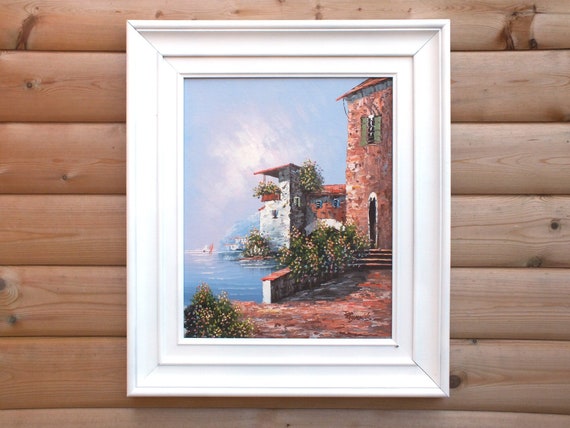This photograph captures a framed painting mounted on a wall of horizontally laid wooden panels, each with a rounded dip enhancing the wooden texture. The frame around the painting is an intricately designed white wooden frame with multiple levels, adding an extra layer of detail to the overall presentation. The artwork itself is an oil painting, possibly depicting a scene from a Mediterranean coastal town. Dominating the foreground is a two-story red stone building with a red roof, bordered by a red sidewalk and a short retaining wall beside the water. The building is beautifully accented by flowering bushes with pink and green hues, both beside it and over the wall. In the painting's background, the sky transitions from darker blues to white and pink clouds, contributing to a serene atmosphere. The blue water near the bottom of the painting features delicate white waves, enhancing the coastal setting. Another white building with flower boxes can be seen in the distance. The artist's signature, beginning with an 'R', is located in the bottom right corner of the painting.